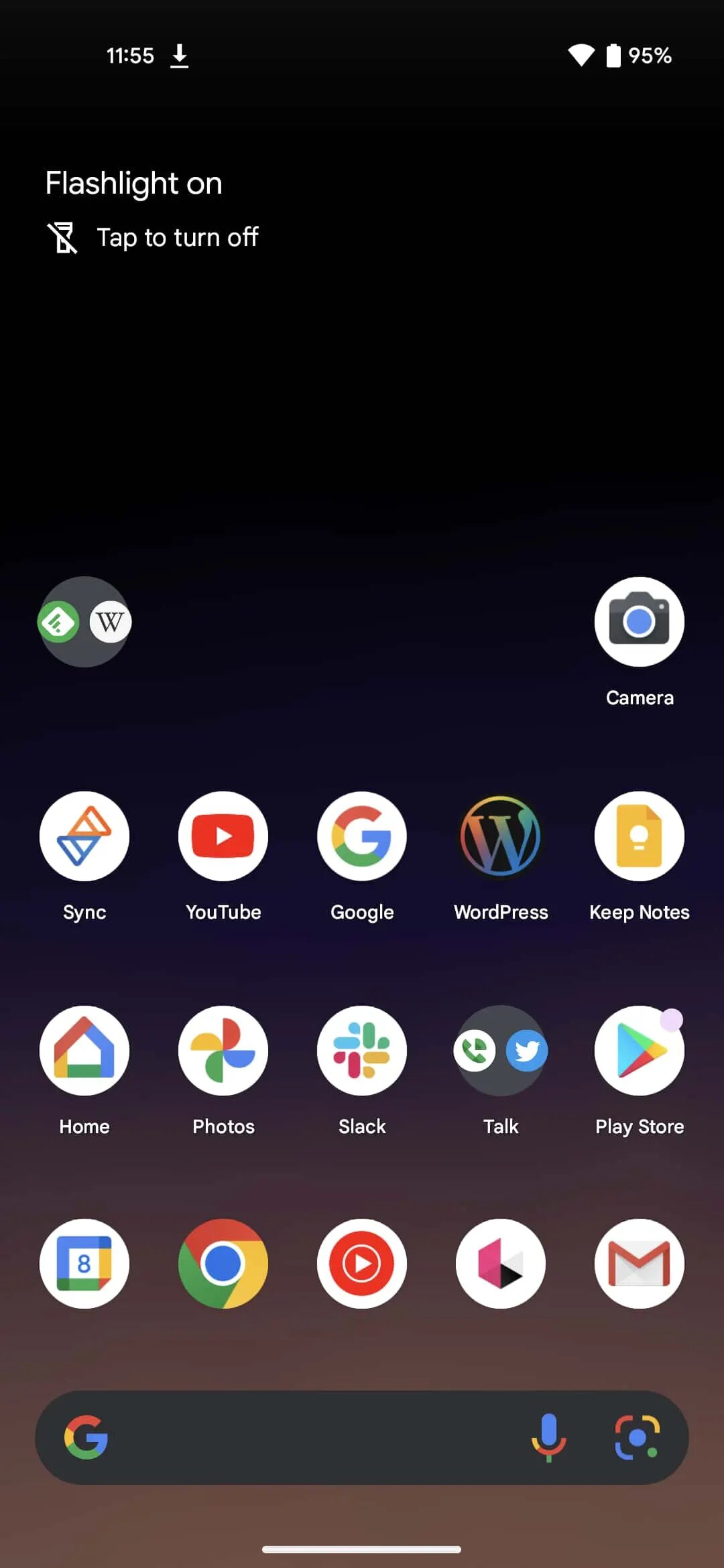A detailed screenshot of a smartphone display taken at 11:55, as indicated by the time prominently shown in the upper left-hand corner of the screen. The image captures the entirety of the phone's interface, including app icons, notifications, and widgets, showcasing a typical smartphone layout at nearly noon. The repetitive nature of the description suggests emphasis on the specific time and the fact that the image is indeed a screenshot, highlighting the importance of these details in understanding the context of the image.